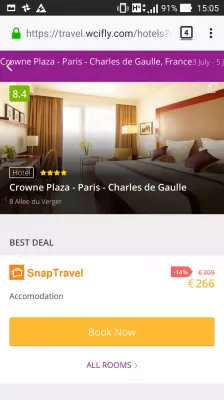This vertical image, likely a screenshot from a smartphone interface, depicts a hotel booking page from a travel website. At the very top, there is a gray status bar with various white icons, including a photo icon, a triangle, and an icon with white lines in various directions, on the left-hand side. On the right-hand side of the status bar, military time reads 15:05, with a battery life of 91%, signal bar strength, and an 'H', followed by an additional icon.

Below the status bar, a lighter gray box contains a green padlock symbol beside the web address. Adjacent to this, three vertical dots indicate more options. Further down, within a purple box, the text "Crowne Plaza, Paris, Charles de Gaulle, France, July 3rd through 5th" is prominently displayed. Below this heading, a green square displays a rating of 8.4. 

A photograph of a hotel room is shown along with the text "Crowne Plaza, Paris, Charles de Gaulle," emphasizing it as the "Best Deal," with “Snaptravel” highlighted in orange underneath. The accommodation offers a 14% discount, bringing the price to £266. Users are presented with an orange "Book Now" button or a purple "All Rooms" button to explore further options.

At the bottom of the image, a medium gray rectangle box concludes the view.